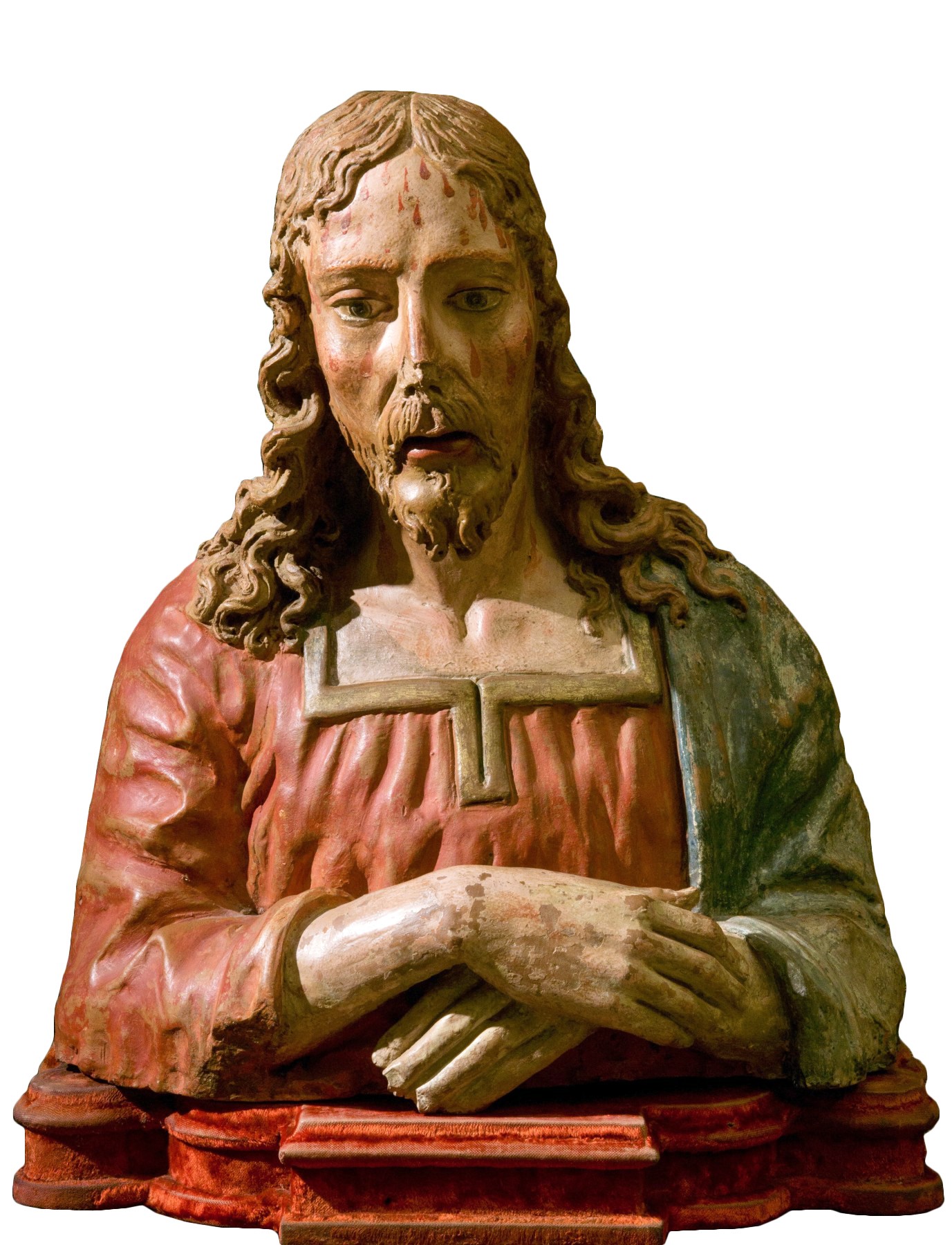This photograph features a detailed and weathered sculpture, presumably of Jesus Christ, set against a stark white background. The statue, capturing Jesus from mid-chest upwards, appears to be crafted from either wood, clay, or possibly plaster, and it has been meticulously painted. His face, marked by a dark grayish beard and mustache, exhibits a pensive expression, with eyes cast downward to the viewer's left and his mouth slightly open. Distinctive blood drops are visible across his forehead and cheeks, reinforcing the depiction of Christ. His long, curly hair flows down to his shoulders. The figure's attire consists of a red robe with gold trim and a greenish-blue fabric draped over his left shoulder, possibly symbolizing a cape or poncho. His hands, rendered with long, detailed fingers, are crossed over his midsection, with his right hand resting on top of his left. The statue is mounted on a thick, red platform, which shows signs of weathering, consistent with the aged appearance of the sculpture.